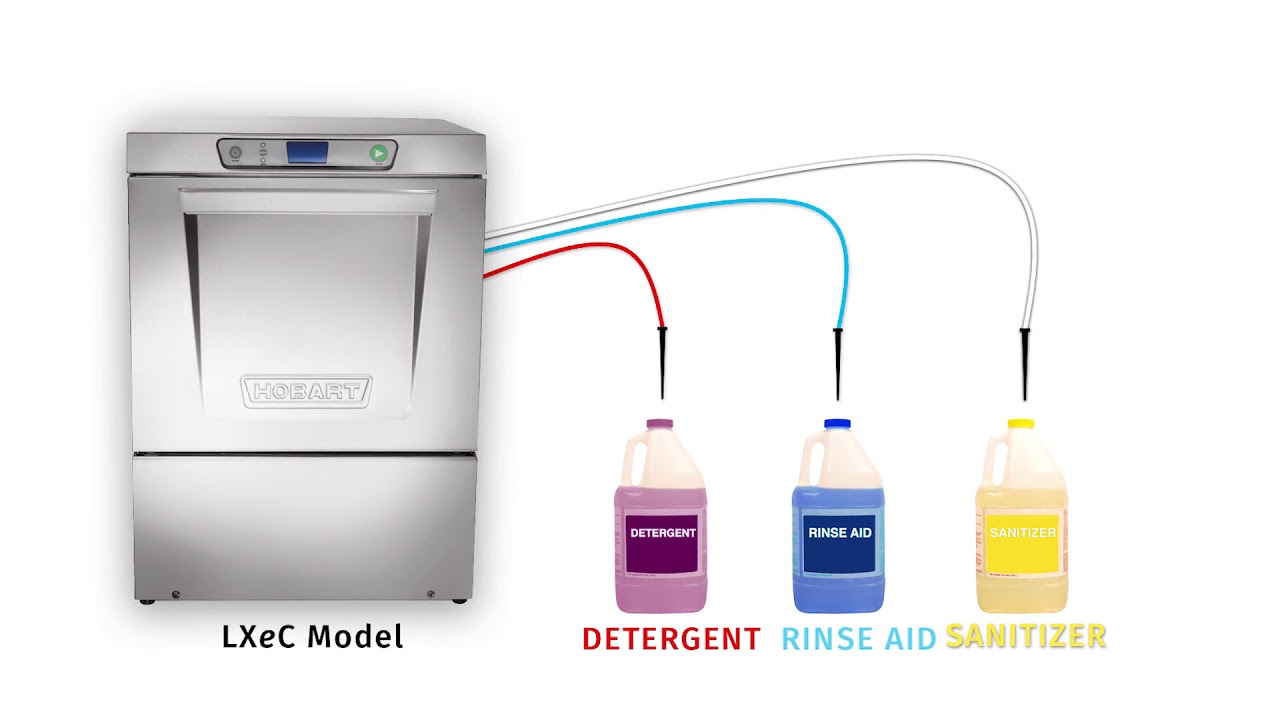The image displays a Hobart LXEC model commercial dishwasher set against a blank white background. Made of stainless steel, the machine features a handle, a display screen, and a green start button at the top, indicating a sophisticated and user-friendly interface. Notably, the door opens towards the user, similar to an oven. On the right side of the dishwasher, three colored hoses extend outward, each connecting to distinct bottles: a red hose to a red detergent bottle, a blue hose to a blue rinse aid bottle, and a yellow hose to a yellow sanitizer bottle. These hoses suggest automatic dispensing of cleaning agents, reinforcing the machine's commercial utility. The setup looks like a catalog or online listing, emphasizing its professional and efficient design.